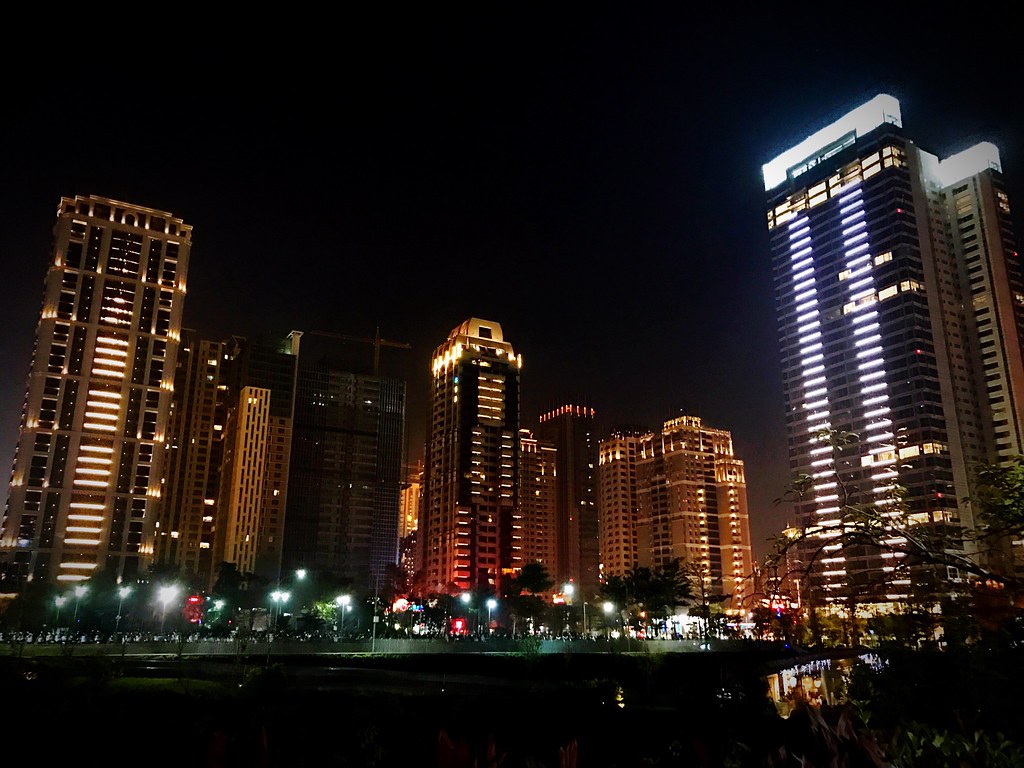This nighttime photograph captures a vibrant downtown cityscape, dominated by approximately nine illuminated skyscrapers. The scene is framed by a pitch-black sky, devoid of stars due to light pollution. The architecture is varied, with lights creating a vertical pattern across the buildings, some floors brightly lit while others remain dark. Prominently in the foreground, seven skyscrapers stand tall with a street running parallel to them, eventually curving slightly to the right. Additional illuminated buildings can be seen at an angle further back. The street is lined with streetlights providing essential illumination for pedestrians. Between the clusters of buildings, a large park area filled with vegetation, including trees and green grass, is visible. Tall poles with large lights ensure the park is well-lit, adding to the overall brightness of the scene. The cityscape is awash in a spectrum of lights, from neon purples to warm yellows and oranges, painting a vivid and dynamic portrait of this urban landscape at night.